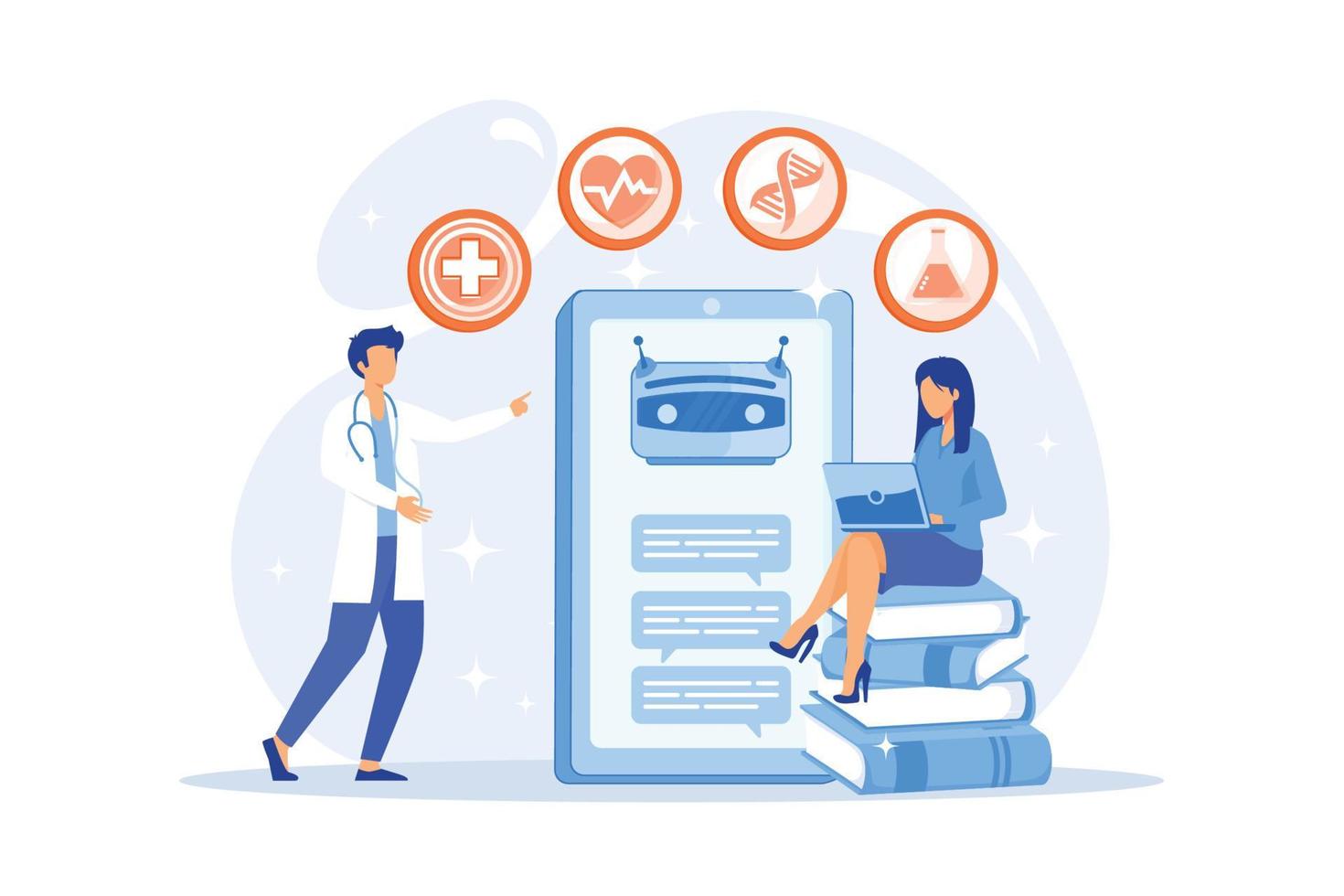In this computer-generated, clip-art-style image set against a light blue, swirly background, a doctor stands on the left of the composition. He has black hair, wears a white lab coat over a gray shirt, black pants, and black shoes. A black and silver stethoscope hangs around his neck. He is pointing at a large, vertically oriented rectangular screen in the center of the scene. The screen has a light blue display with a blue border, showing the top of a robot's head and three conversation bubbles beneath it. 

To the right of this screen, a woman sits cross-legged on a stack of four blue books with striped spines. She has black hair and wears a dark blue skirt, a light blue button-down shirt, and blue high heels. On her lap is a light blue laptop. Her facial features are drawn in a simplistic, cartoon-like style.

Above the screen are four circular health-related icons in reddish hues. From left to right, they depict a medical cross, a heart with EKG lines, a DNA helix, and a beaker partially filled with an orange liquid. The entire image blends various shades of blue and includes elements in red, creating a cohesive, visually engaging scene.